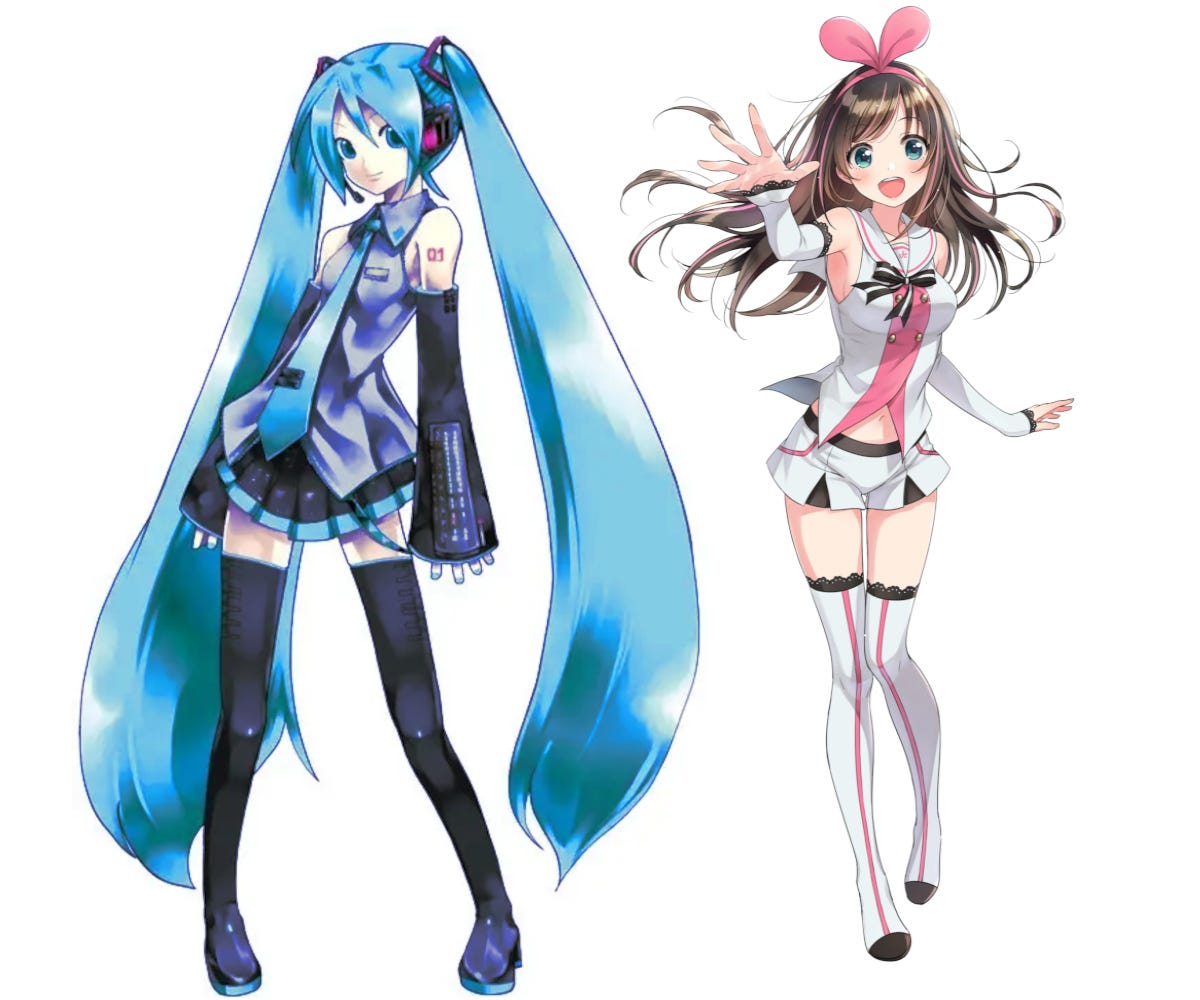This image features two anime characters set against a plain white background. On the left is a girl with extraordinarily long blue pigtails that reach her feet, styled in high ponytails with wispy bangs. She wears a short-sleeved button-up shirt featuring a blue tie and a short skirt that alternates between blue and black. Black arm coverings flare out from her sleeves, revealing only her fingers, and she has long black thigh-high socks. Her futuristic appearance is augmented by a tattoo marked "01" on her left shoulder and a pink headset.

On the right stands another girl, distinguishable by her pink bunny ears and long brown hair that cascades to her shoulders. She reaches out towards the viewer, dressed in a short-sleeved white button-up shirt adorned with a red bow in her hair, a pink inner shirt, and gold buttons. Her outfit includes white lace arm coverings extending to her palms, a skimpy white skirt that mirrors the colors of her knee-high socks, trimmed with black lace and featuring pink stripes and brown accents at the toes and tops. Both characters exude a youthful, vibrant aesthetic, likely between the ages of 14 to 16, and are designed with meticulous detail, emphasizing their distinct yet complementary styles.